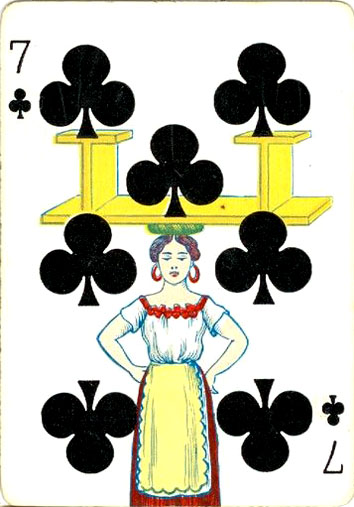The image features a distinctive playing card with an ornate design. The card showcased is the Seven of Clubs, highlighted by a thin golden outline along its edges. The top-left and bottom-right corners display the black "7 ♣" symbol, oriented in their respective standard and upside-down positions. Central to the card’s layout, seven club symbols are arranged in three columns: three clubs in the first column, one club in the second, and three more clubs in the third.

Dominating the center of the card is an illustration of a woman dressed in traditional Spanish-inspired attire. She wears a white short-sleeved blouse adorned with a red floral border at the neckline. Large red hoop earrings accessorize her ensemble, complementing her neatly parted brown hair, which is tied back. Atop her head rests a flat yellow board, ornamented with two "T" shapes on either side.

Her outfit is completed by a long, flowing red skirt. Over the skirt, she dons a yellow apron with a scalloped edge that cascades elegantly from her waist. The rich colors and detailed costume bring a vibrant, cultural charm to the card, making it a unique piece within the deck.